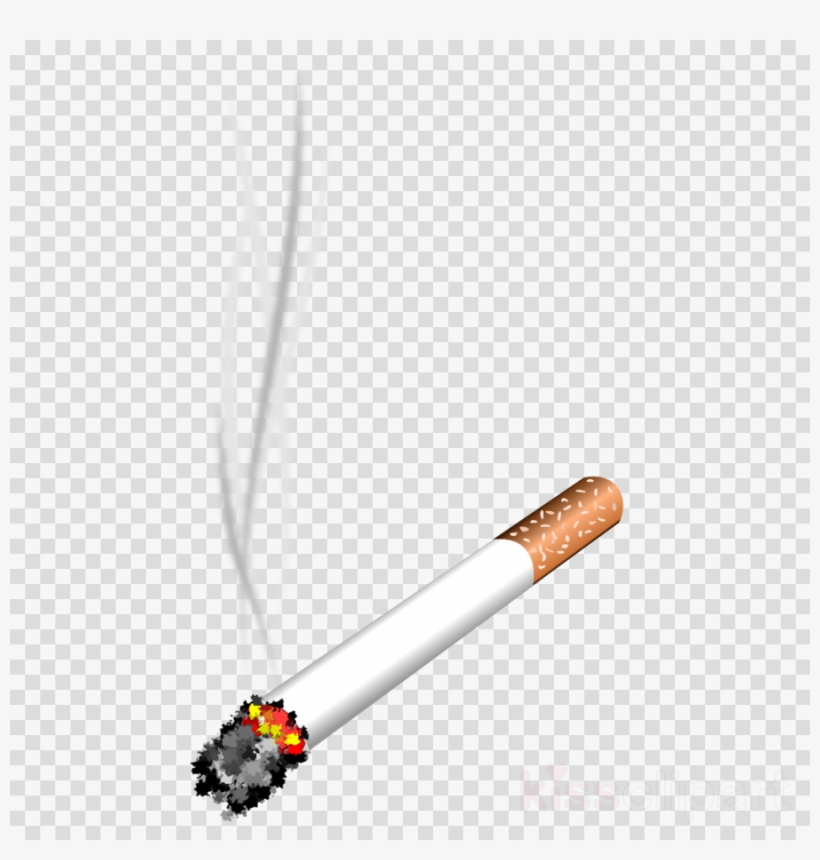The image is a digital illustration, likely created by a graphic designer using a simple program like Windows Paint. It features a lit cigarette positioned diagonally from the bottom left to the top right of the page against a gray and white checkered background, indicative of transparency. The cigarette includes a detailed depiction of the white cylindrical paper, the brown speckled filter, and the burning cherry, with hues of orange and yellow. Ash is accumulating at the bottom left of the page. Smoke billows and curls up from the lit end, extending towards the top of the image in various shades of gray. The illustration employs gradient shading to give the cigarette a contoured appearance.